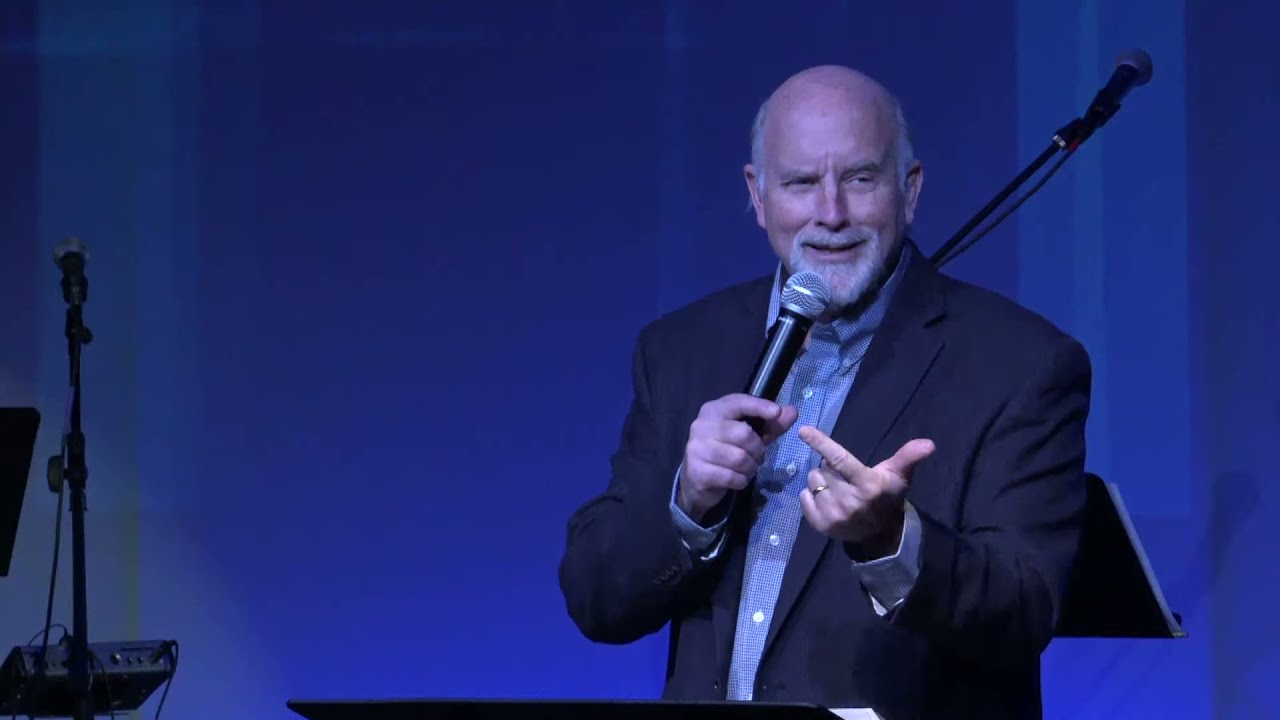The image depicts an older white man, likely in his late 60s to early 70s, who appears to be giving a presentation or speech in a room with a prominent blue background. He has a mostly bald head with some white hair on the sides, and sports a white mustache-goatee combo. Dressed in a blue suit jacket and a light blue button-down shirt, he holds a microphone close to his mouth with a slight smile, suggesting he's in mid-speech. His body is angled slightly to the left while his head is tilted a bit to the right. He makes a gesture with his free hand, thumb and index finger extended, and wears a gold ring on his finger. Beside and behind him are various pieces of audio equipment, including another microphone that is placed higher than his head, and a black podium with a music stand holding papers, hinting at a possible performance or religious event. The overall scene has a distinct blue hue with a combination of audio devices indicating a well-planned setup for speaking to an audience.